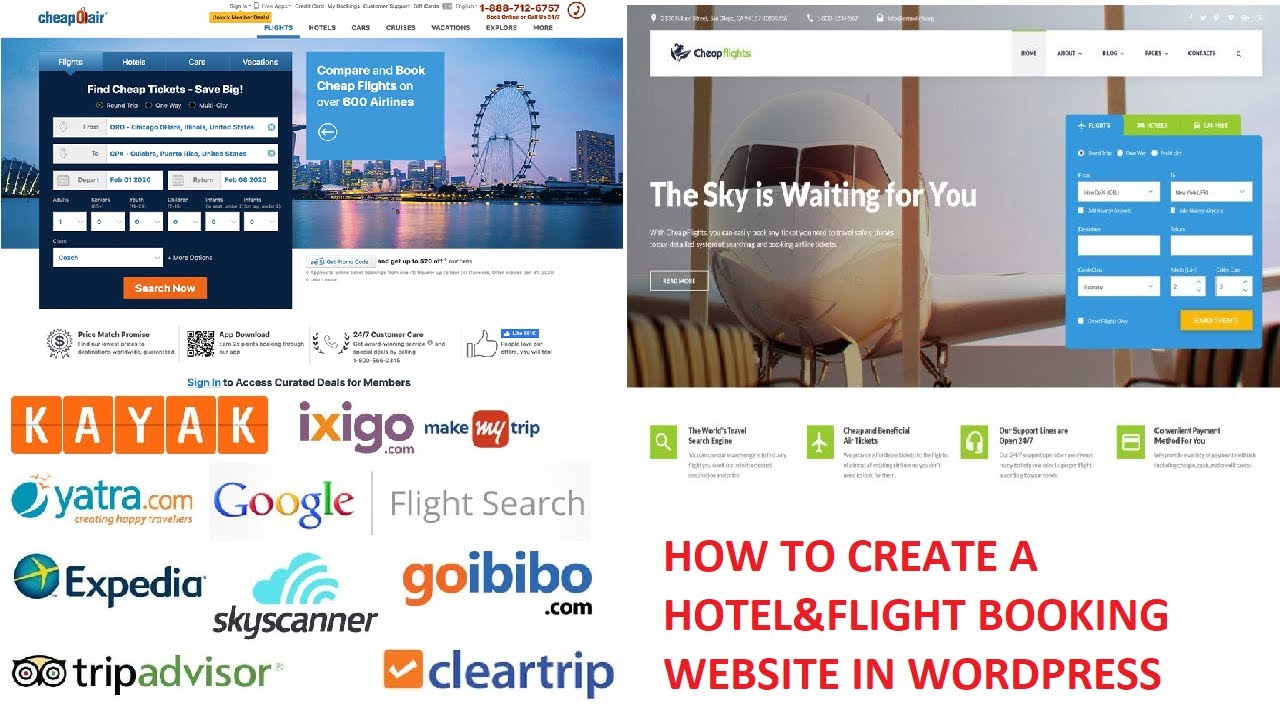The digital image depicts an online travel website with a clean white background, elegantly divided into two distinct sections.

On the right side of the screen is the "Cheap Air" section. The distinctive Cheap Air logo is prominently placed in the corner, alongside a streamlined text menu bar for easy navigation, and a contact number for customer support. A vibrant color illustration of an entertainment area on a waterway, featuring a visible Ferris wheel, serves as the backdrop. Superimposed on this illustration is a data screen titled "Find Cheap Tickets, Save Big." Within this screen, users can enter various search parameters to find travel tickets. Below the data entry points, the website highlights four key factors that define its service. A row of recognizable company logos such as Expedia, Kayak, Google, and TripAdvisor underscores their wide-ranging integrations and partnerships.

On the left side is the "Cheap Flights" section. It features a captivating color image taken from an airport terminal, looking through large glass windows at a plane ready for departure. Bold white text across the image reads, "The sky is waving for you," enticing users with the allure of travel. Adjacent to this image is a small blue window with fields to input search parameters for flight tickets. Below this input area, four separate sections of text accompanied by green icons detail the various features and benefits that Cheap Flights offers. At the bottom of the left side, large red letters announce, "How to create a hotel and flight booking website in WordPress," providing guidance for those interested in developing a similar platform.